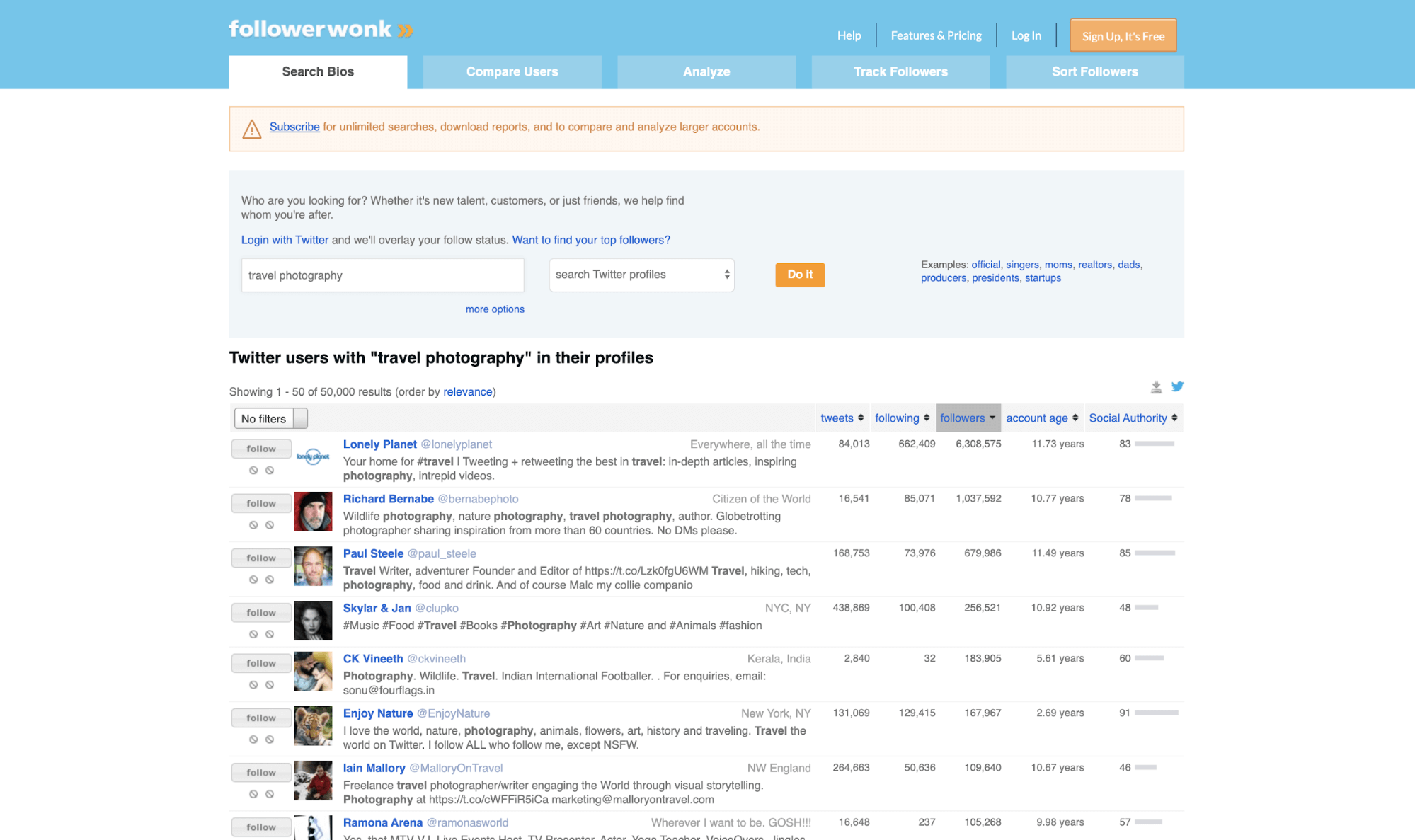The image features a website interface set against a light blue background. 

At the top, there is a large blue banner with the text "Followerwonk" accompanied by two small orange arrows pointing to the right. Below the banner, a set of tabs is visible, including a prominent white tab labeled "Search." 

Further down, the interface contains multiple blue boxes and descriptions. Seven blue boxes are organized as follows: three at the top, followed by four below them. Additionally, there is an orange box positioned among these blue boxes. 

Directly beneath the search tab, a pink box has appeared with a red triangle icon and an exclamation point, containing a "Subscribe" message and associated information.

The main content area contains another blue box with finely printed text describing options like "Log in with Twitter." The interface allows users to log in and search Twitter profiles via a white input box labeled for this purpose. Adjacent to this, a small red button labeled "Do It" is displayed. 

To the right of the input box, the text "Twitter users with travel photography in their profiles" is displayed along with additional descriptive text. Below the header, there is a blue box labeled "Mac users" and a series of user listings. 

Each listing includes a user’s picture and symbols, possibly stars or dots, in front of their names. Notable users listed are from Lonely Planet, Richard Barnaby (leaning towards Barnaby), Paul Steele, Skyler, Jan, CK, and another user labeled "Enjoy Nature." Each user has comprehensive stats displayed to the right of their names and photos.